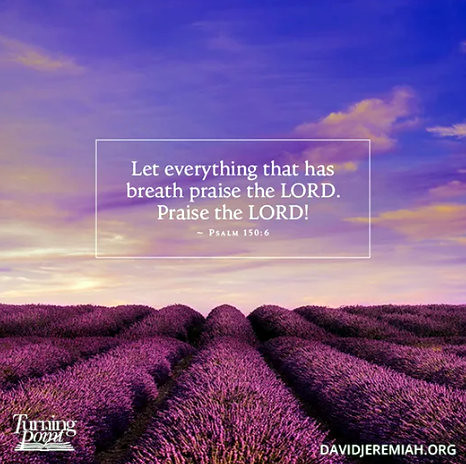This vertical rectangular image appears to be a religious poster featuring a visually striking background. The sky, a blend of blue, purple, and white, has an artificially colored, photograph-like quality with soft, white clouds. Below the sky lies a vast field covered in dark purple crops, creating a surreal and serene landscape. Centered within the image, a white rectangular text box prominently displays the verse, "Let everything that has breath praise the Lord. Praise the Lord. Psalm 150:6," written in white letters. The lower left corner of the image bears the logo "Turning Point" in white text, while the lower right corner features the URL "davidjeremiah.org," also in white text.